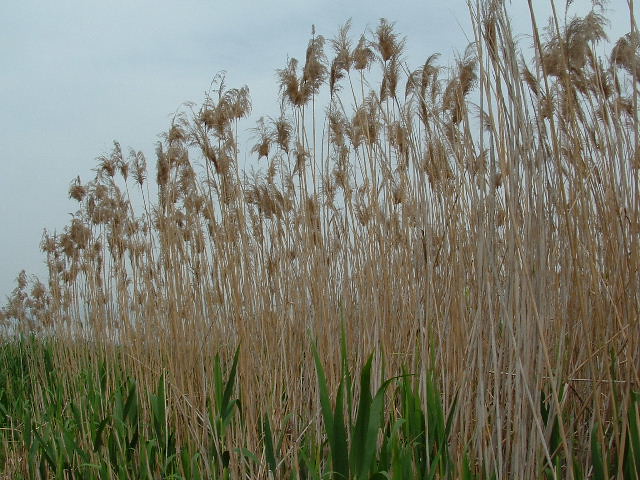This is a detailed outdoor daytime photo showcasing a natural scene with no people or text. Dominating the picture are tall, brown stalks of plants, topped with fuzzy brown tips, rising prominently from left to right. These stalks, which resemble dry hay or weeds, are notably much taller than the plants in the foreground. The foreground features a different type of flora: long, tapered green leaves akin to blades of grass, reminiscent of corn leaves. These green blades provide a stark contrast to the dense cluster of brown stalks. In the upper part of the image, the sky appears overcast, with a light gray or light blue hue, creating a muted and cloudy backdrop. The entire scene conveys a sense of natural simplicity, with the tall dry plants standing out against the green leaves and the softly colored sky.